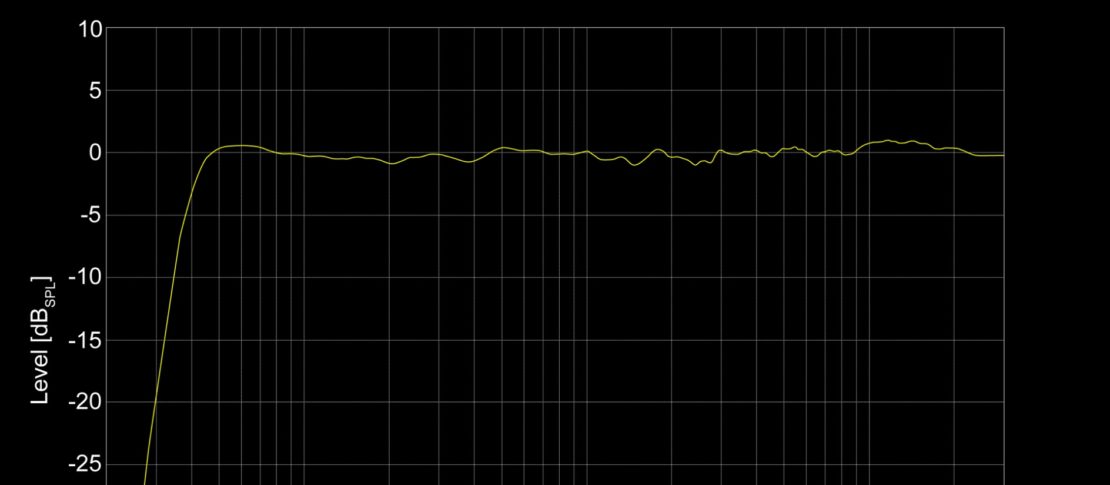The image features a black background with a detailed graph superimposed on it. Along the left side of the graph, there is a vertical axis labeled "Level" with numerical markers at intervals of 5, ranging from 10 at the top to -20 at the bottom. The graph is segmented by numerous vertical and horizontal grid lines that span across the entire page, creating an intricate lattice structure. Prominently, a green line traverses from one end of the graph to the other, dynamically fluctuating in height according to the specific levels indicated on the vertical axis, ranging between values such as minus 5, minus 10, and others. This green line captures the varying data points across the graph, illustrating the changes in level as it moves horizontally.